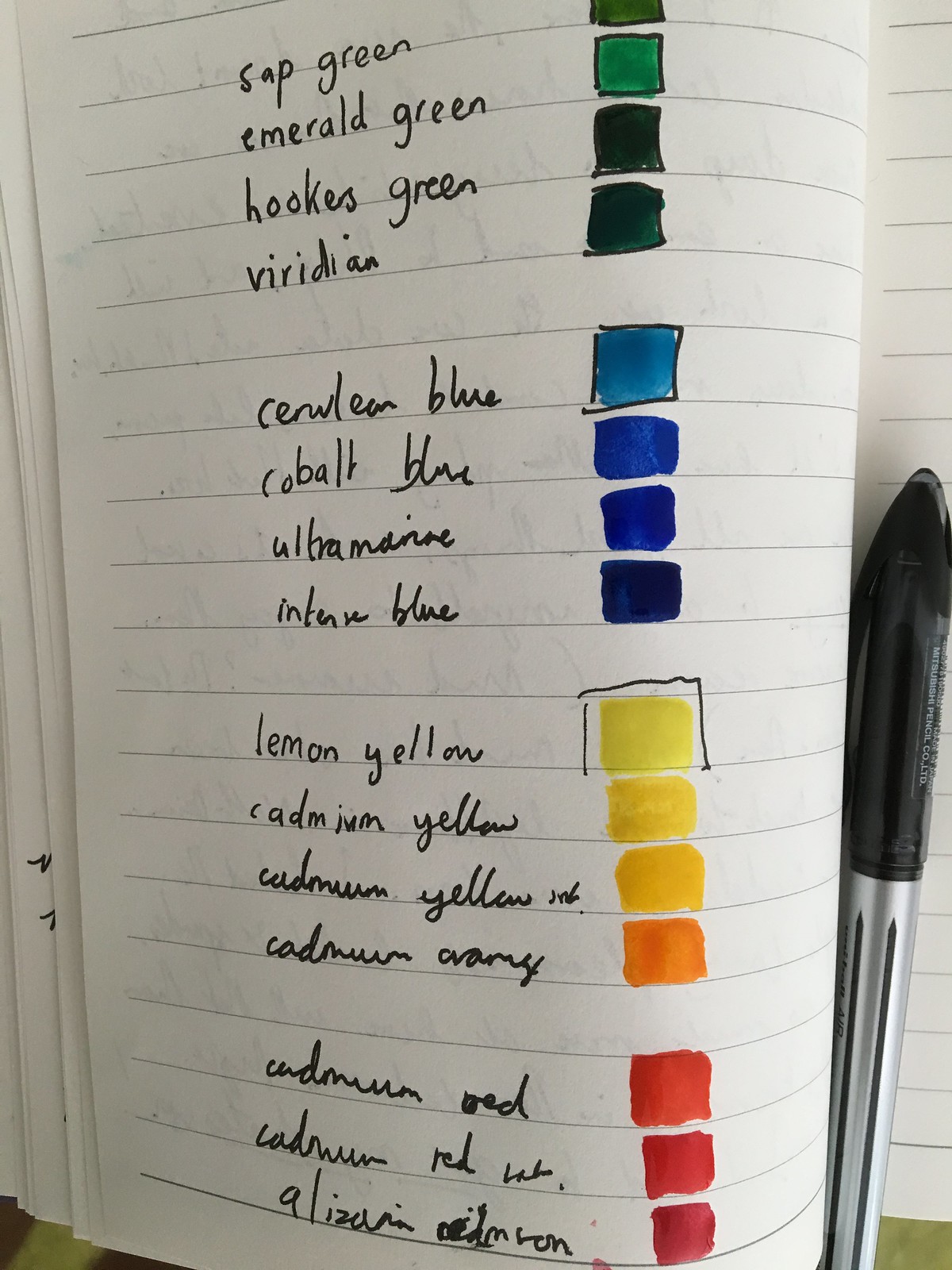The image captures a photograph of a lined white paper notebook. On the right side of the open page, there are approximately 17 rectangles sketched out in different colors, transitioning from various shades of green at the top to blues, then yellows, oranges, and finally reds toward the bottom. Each rectangle is meticulously labeled with the corresponding color name written on the left side of the page. The shades include names such as sap green, emerald green, hooker's green, viridian, cobalt blue, cerulean blue, ultramarine, indigo, lemon yellow, cadmium yellow, and cadmium red among others, although some labels near the bottom edge are hard to decipher. Additionally, there is a pen with a black cap positioned on the right side of the notebook, contributing to the artistic and organized presentation of the color swatches.